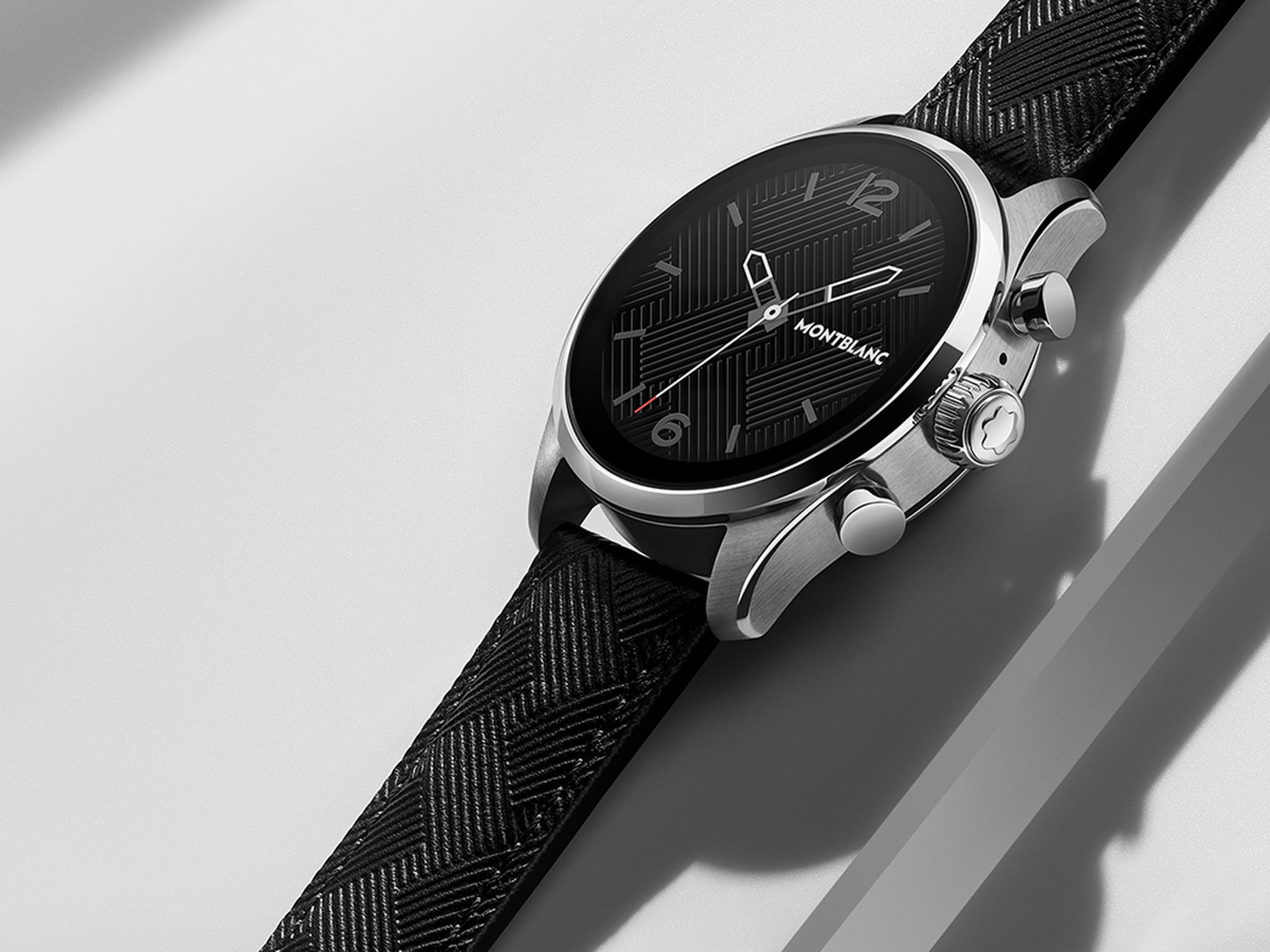This up-close, highly-detailed image of a watch on a sleek white table captures the luxurious essence of a Montblanc timepiece, suggestive of being suitable for a young professional or businessman. The watch boasts a textured black strap adorned with a crosshatch pattern, mirroring the intricate design on its black face. The face of the watch features two prominent numerals, ‘12’ and ‘6’, with slim, gray lines for the remaining hour markers. The hands of the watch, outlined in white, appear distinctly against the black background, adding a modern touch to the overall aesthetics. Encased in shiny, metallic silver, the watch's edge and three rotary knobs enhance its sophisticated look. The image, whether a high-quality photograph or a computer-generated render, effectively highlights the blend of sleek design and luxurious craftsmanship that Montblanc is known for.